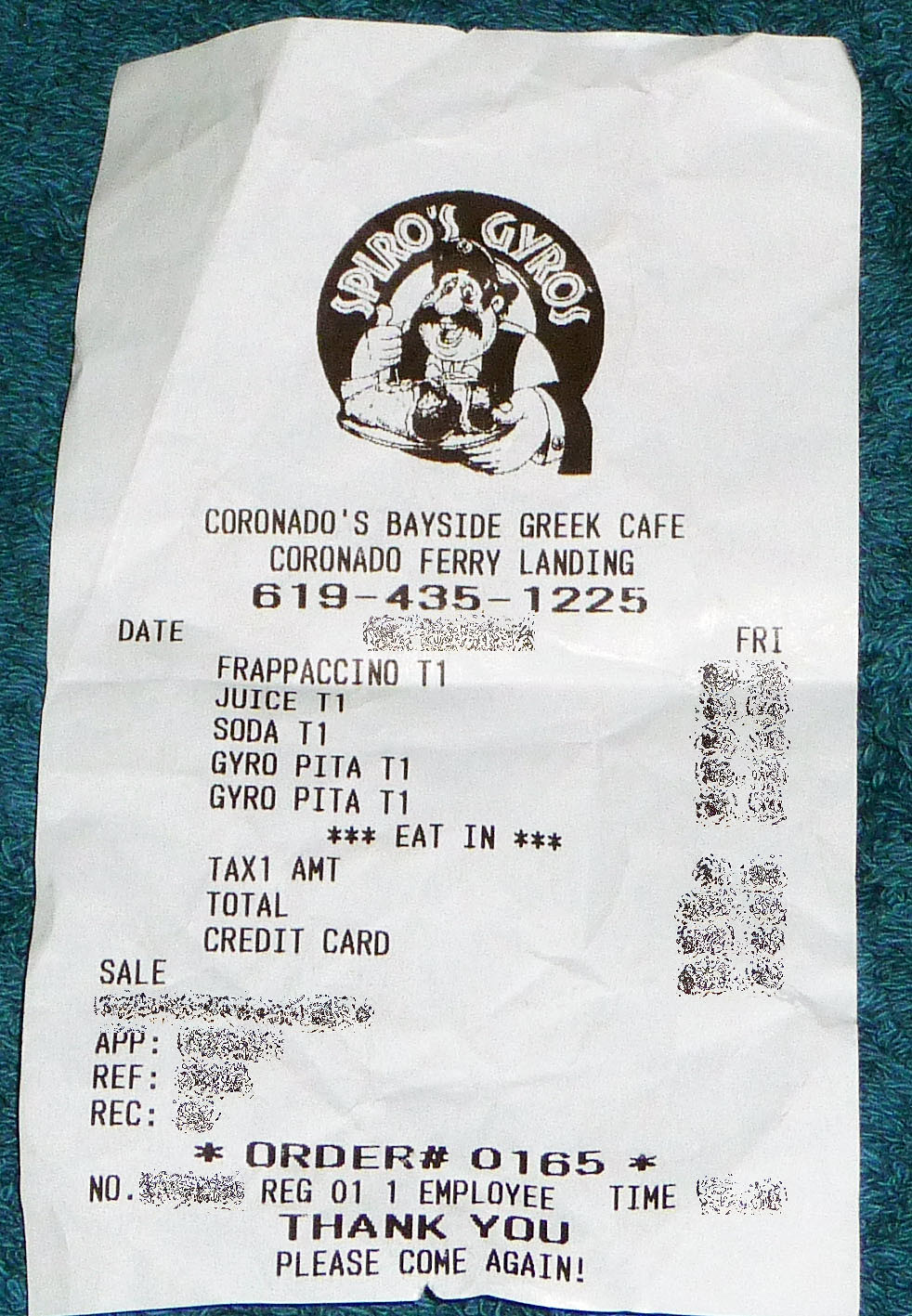A crumpled receipt from Spyro's Gyros, a Greek restaurant, lays atop a handwoven teal cloth table covering. The receipt features the restaurant's logo, depicting a man with a thick mustache, wearing a hat, black vest, and long white sleeves, enjoying a plate of gyros. The establishment, identified as Coronado’s Bayside Greek Cafe located at Coronado Ferry Landing, lists their contact number as 619-435-1225. Although the exact date is blurred, it is noted that the purchase was made on a Friday. The receipt itemizes various orders including a Frappuccino, juice, soda, and two Gyropitas, each with the price details obscured. It mentions the service as eat-in, with sections for tax amount, total cost, and payment via credit card all blurred out. An order number 0165 is marked with an asterisk, alongside additional numbers and codes that are illegible. The bottom of the receipt concludes with a friendly note: “Thank you, please come again.”